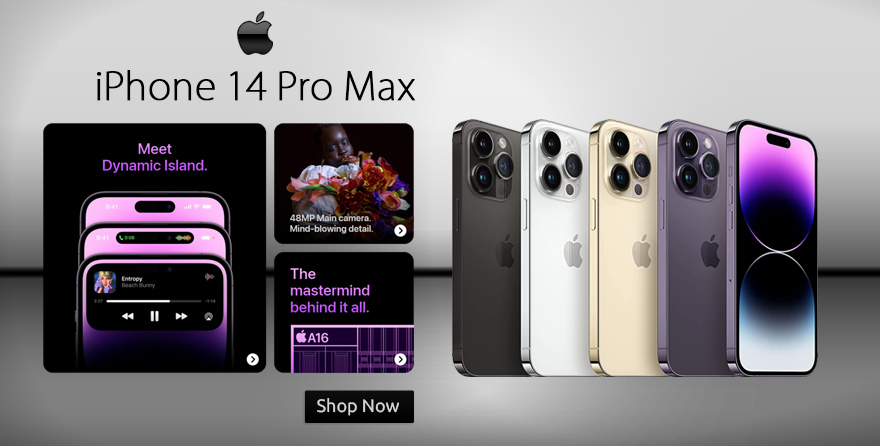This advertisement image for the iPhone 14 Pro Max showcases a visually striking array of five phones arranged in an accordion style on the right side of the page. The lineup includes various color options, beginning with an all-black model, followed by a white one, a cream-colored one, a silverish purple variant, and finally one phone displaying the front view. The iPhone 14 Pro Max prominently features three rear camera lenses and a distinctive clear sensor area. The front view of the phone reveals a vibrant screen illuminated in a gradient of purple and pink at the top, transitioning to black in the middle, and ending with hues of white and green at the bottom.

On the left side of the image, the branding is prominently displayed with the Apple logo at the top. Below it, there is text introducing the "Dynamic Island" feature. A highlighted box states "the mastermind behind it all," referring to the powerful A16 chip. Additionally, the ad emphasizes the phone's advanced photography capabilities with a note that reads, "48MP main camera, mind-blowing detail."